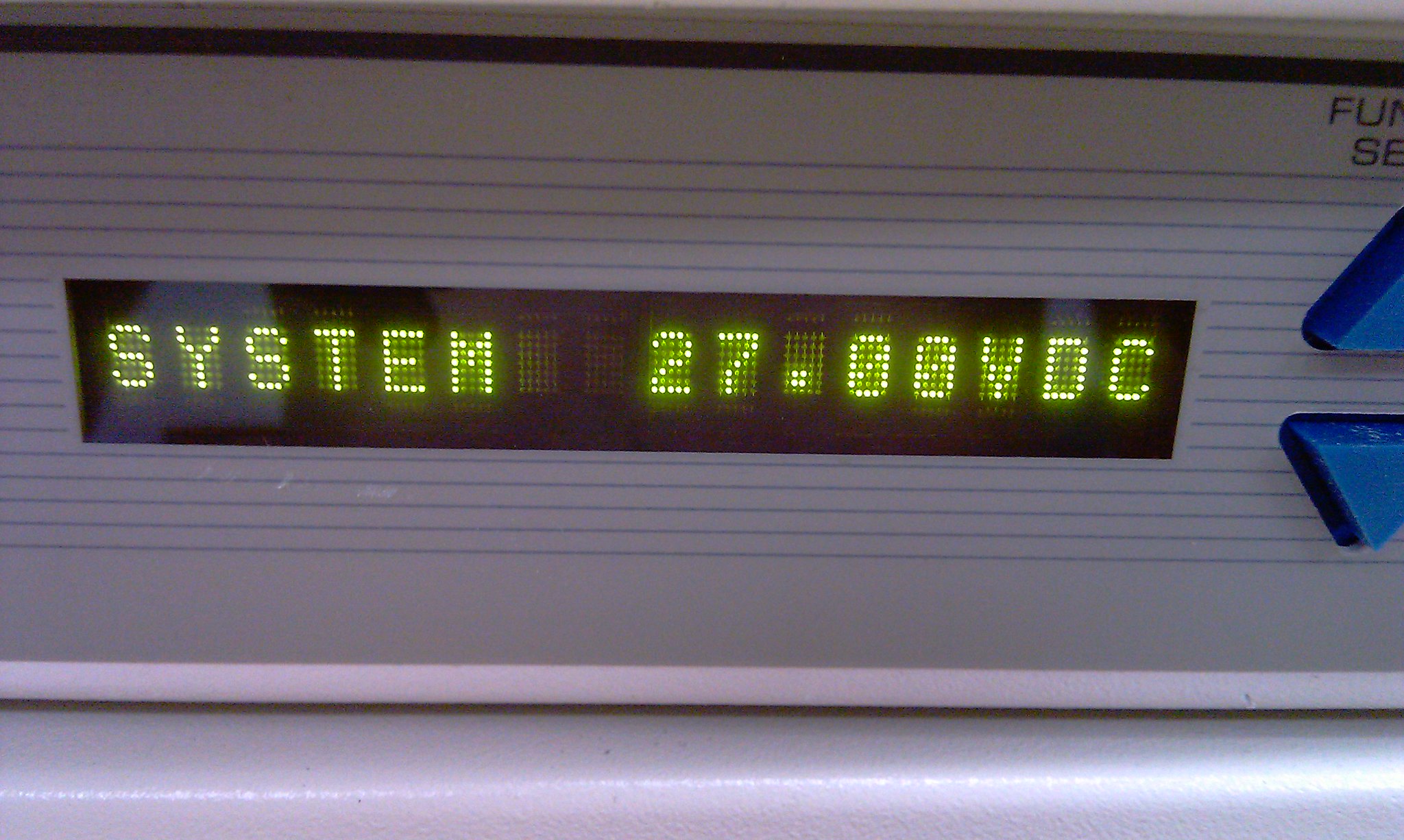This image depicts an electronic control device designed with a sleek white exterior, accented by horizontal blue stripes. On the right side of the device, there are partial and unreadable text markings. Prominently featured are two blue buttons, one with an upward-pointing arrow and the other with a downward-pointing arrow, likely used for adjusting settings. Centrally located on the device is a digital screen, displaying the text "System 27.00 VDC" in bright green characters against a black background, indicating a voltage reading. Overall, the control panel combines functional design with clear, legible output for user interaction.